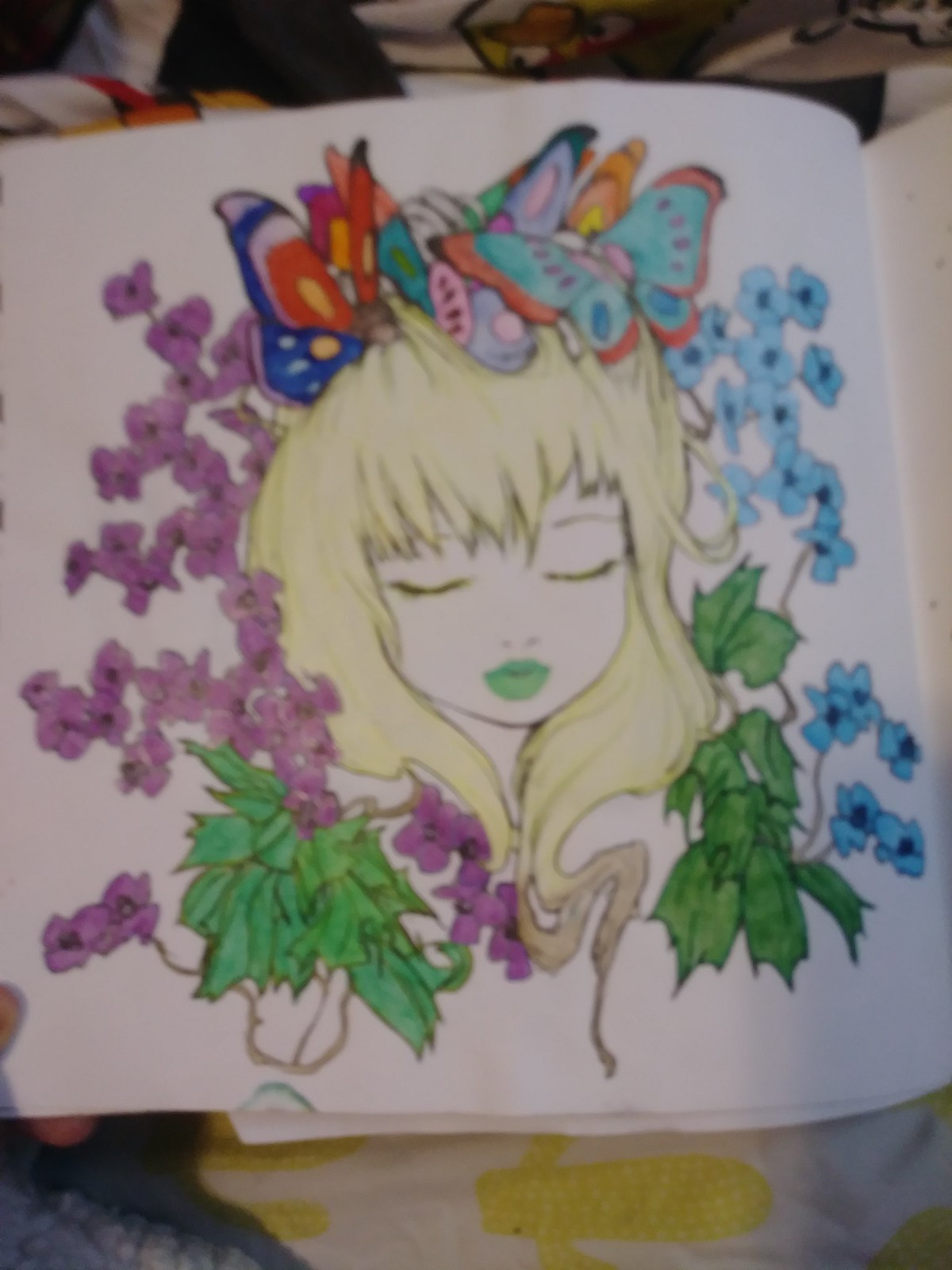The image is a detailed, cartoonish drawing—possibly from a sketchbook or coloring book—depicting a close-up of a girl's face with pronounced, overly large eyes, a small nose, and pouty green lips. Her hair is a faint yellow color, cascading around her face and partially covering her neck, with long bangs obscuring one of her eyebrows. The girl’s head is adorned with a cluster of colorful butterflies of varying hues, including blue, red, orange, lavender, pink, white, black, yellow, and orange. Surrounding her face are a mix of blue flowers on the right and purple flowers on the left, each accompanied by green leaves. The drawing is outlined in a consistent black line. The background includes yellow cactus designs on white, and the edge of what appears to be a bed sheet. In the bottom left of the image, the fingers of the person holding the sketchbook are visible.